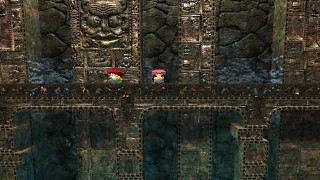In this pixelated game image, which harkens back to classic, low-resolution graphics, two characters reminiscent of LEGO figures stand on a bridge. The setting appears to be within a dungeon or an ancient ruin, emphasizing an atmosphere of mystery and antiquity. The surrounding walls are adorned with artistic faces, perhaps representing the ancient inhabitants or deities associated with these ruins. The bridge they are on is detailed with pillars, and its trim features distinctive black rectangular accents, enhancing the sense of architectural history and depth.